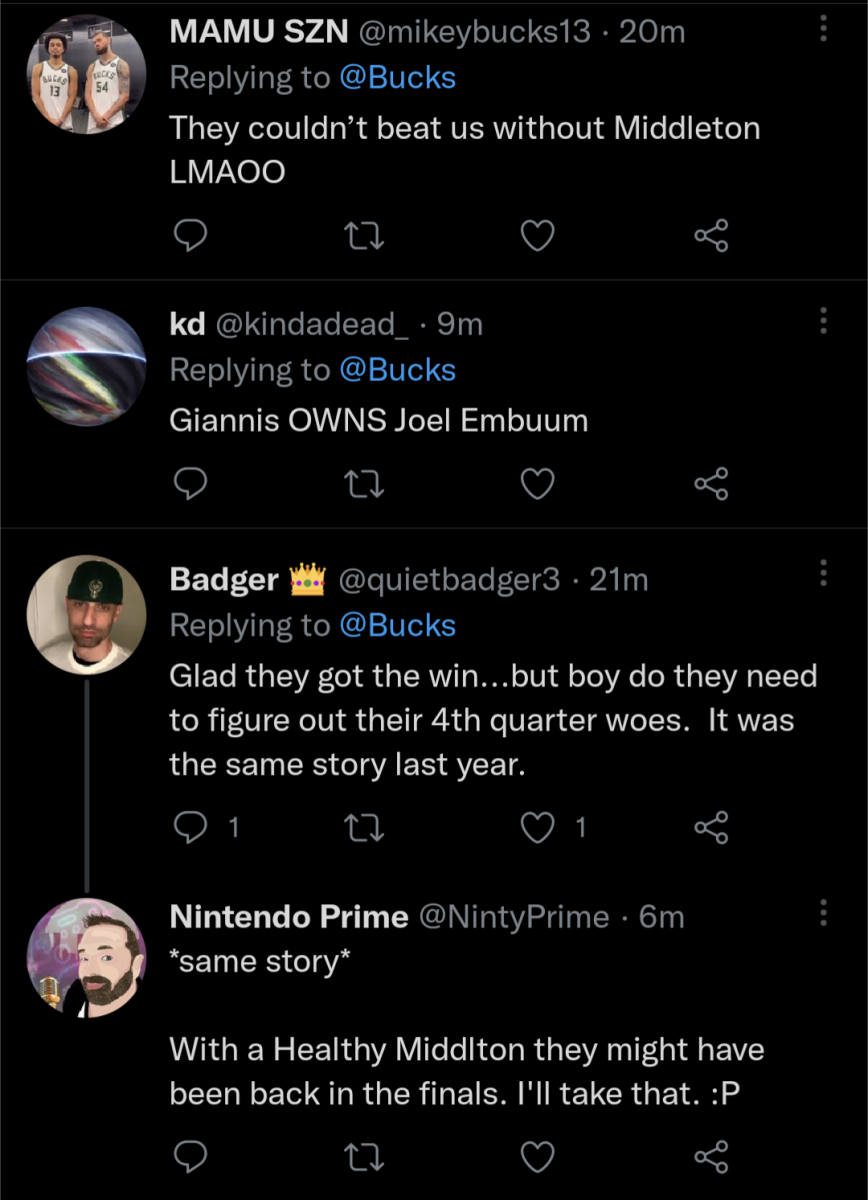The image is a screenshot from a social media platform, likely Twitter, showcasing a thread of replies to the username @Bucks, the handle for the Milwaukee Bucks basketball team. The background is black, and each post is accompanied by the user's profile picture in small circular icons to the left. 

1. The top comment is from the user "MamuSeason," who wrote: "They couldn't beat us without Middleton, LMAOO," with the final word in uppercase.
2. Below that, a user named "KD" (in lowercase) commented: "Giannis OWNS Joel Embiid," emphatically capitalizing "OWNS."
3. The next reply is from a user named "Badger," identified by a crown emoji next to their name, who stated: "Glad they got the win. But boy, do they need to figure out their fourth quarter woes. It was the same story last year."

These comments reflect fans' reactions to a recent basketball game, specifically discussing the Milwaukee Bucks team and their performance, with particular focus on players’ contributions and game strategies.